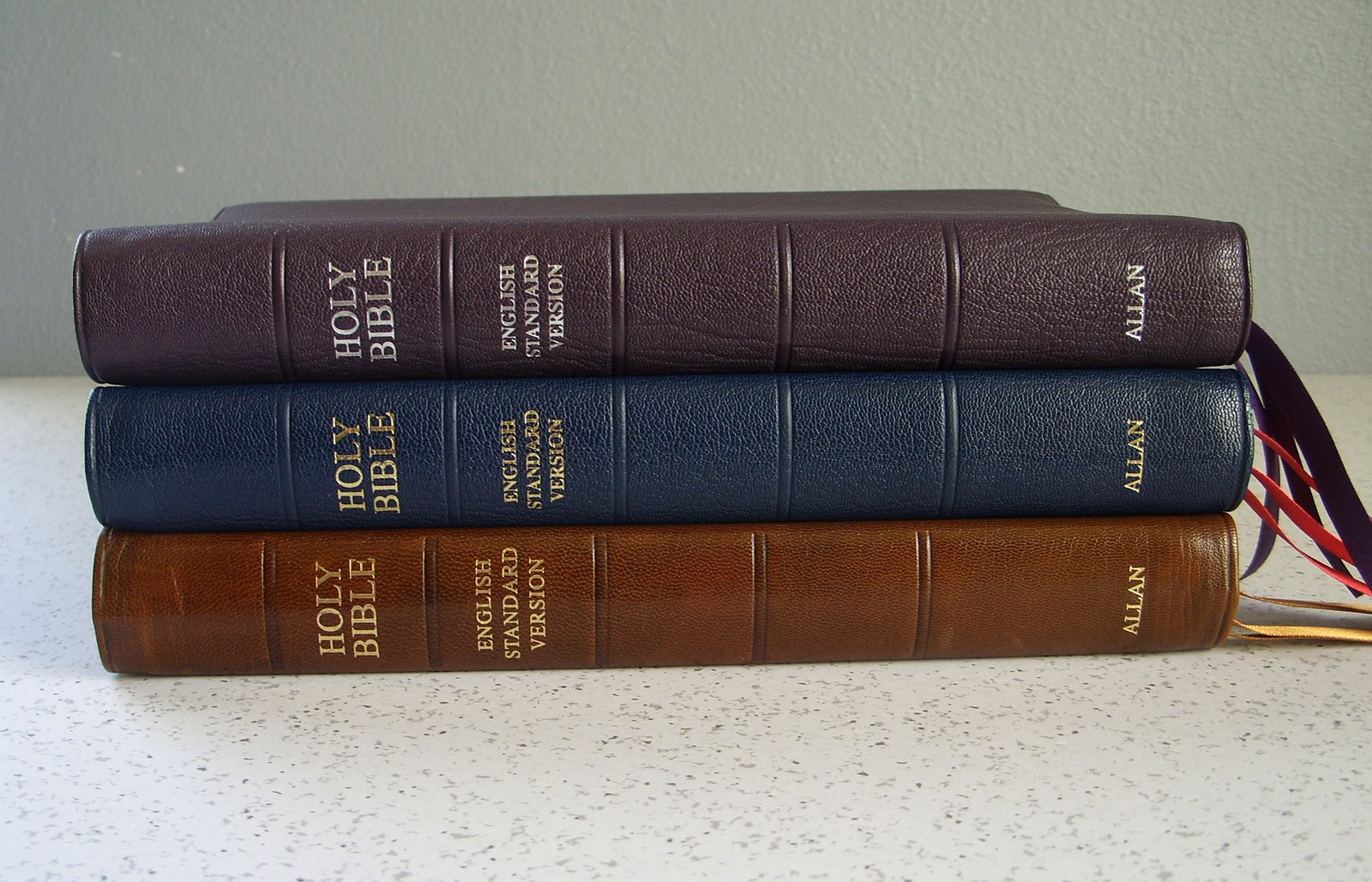This color photograph features a stack of three Holy Bibles, English Standard Version, published by Allen (A-L-L-A-N). Each Bible is leather-bound in differing shades: the top one is light brown with gold text and gold ribbons, the middle one is dark blue with gold text and red ribbons, and the bottom one is chocolate brown with gold text and chocolate brown ribbons. The Bibles, which are identical in size and make, rest on a white marble countertop accented with black and light gray specks. The background is a cream-colored wall that appears almost light gray due to the lighting. Each Bible prominently displays "Holy Bible" in gold text and has multiple ribbon bookmarks extending towards the right. The detailed textures of the leather covers and the sheen of the metallic text and ribbons add richness to the composition.